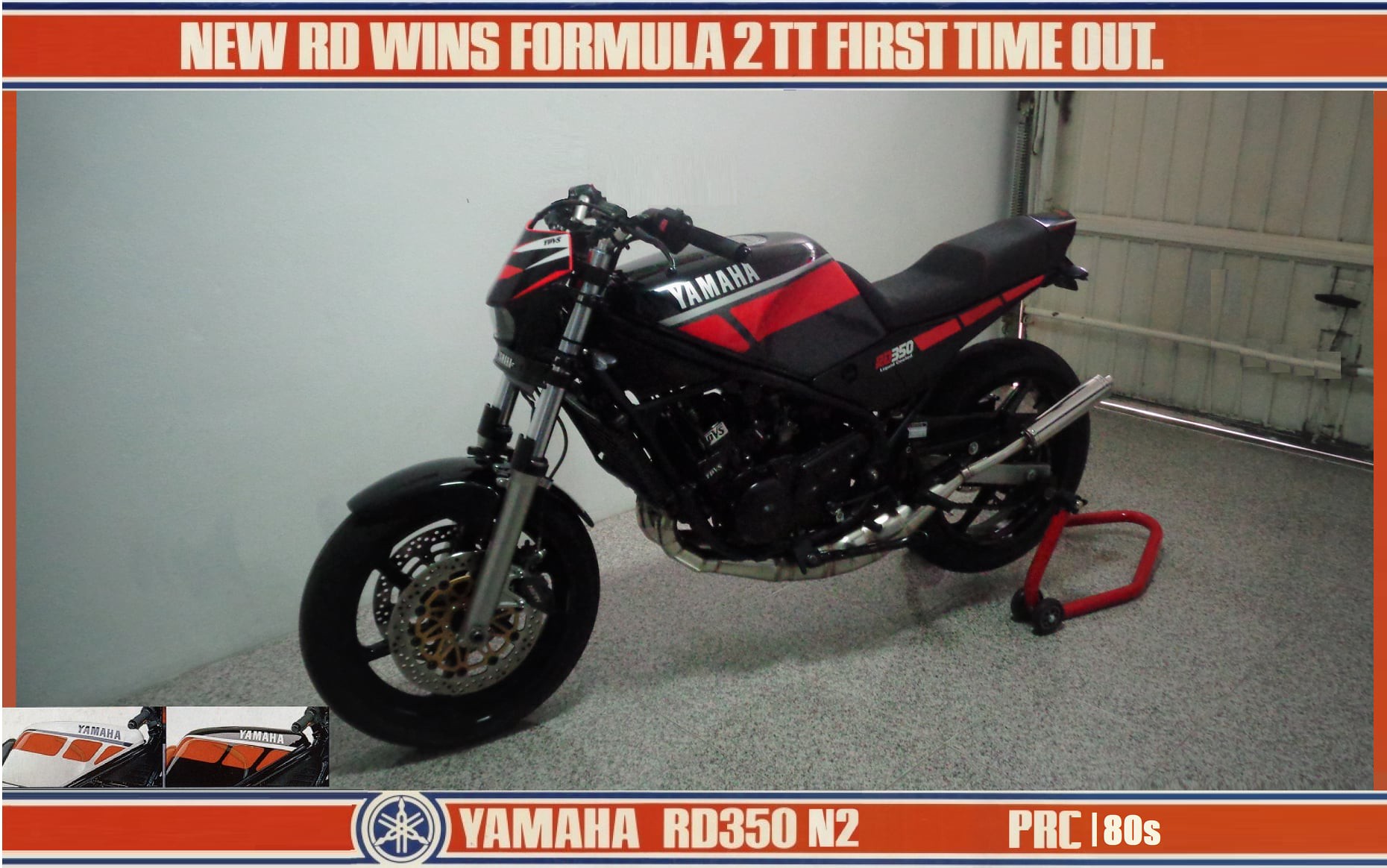The photorealistic image showcases a Yamaha motorcycle prominently in the center, facing slightly to the left. The motorcycle is adorned in a striking black and red color scheme, with a predominantly black body accented by red designs. The word "Yamaha" is emblazoned in silver lettering on the motorcycle's central body. Anchored at the rear, a supportive red contraption made of plastic or metal is visible.

The setting appears to be a garage or shop, with the motorcycle positioned on a composite ground that is white speckled with various colors. The background features a white wall and a closed white garage door on the right side of the image. 

A distinct border of red, blue, and white frames the image. At the top, a red banner with white text proclaims, "New RD Wins Formula 2 TT First Time Out." At the bottom, another red banner includes a Yamaha logo near the left-middle, followed by the text "Yamaha RD 350 N2" and "PRC line 80s" further right. In the bottom-left corner, there are small pictures of two versions of the motorcycle's body: one in white and red, and the other in black and red.